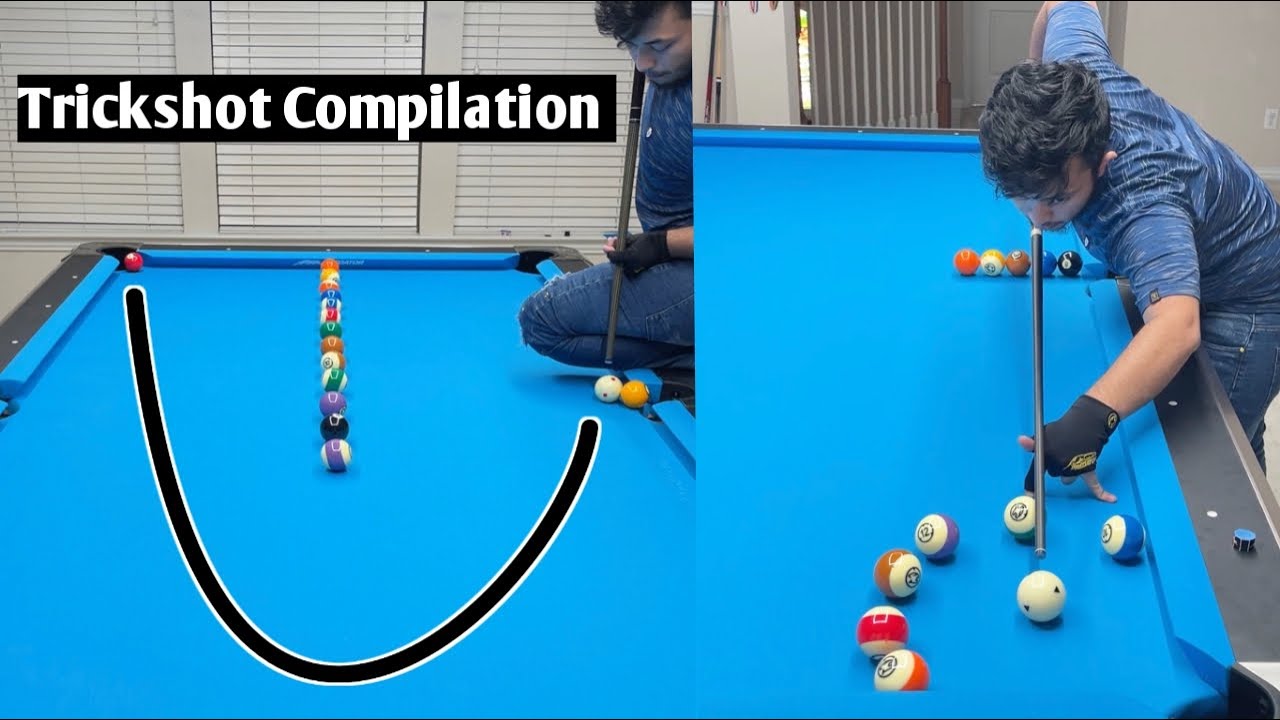In this rectangular image, two photographs are displayed side by side, both featuring the same man performing trick shots on a bright blue pool table with black wooden rails. 

The photograph on the left showcases a man in his 20s, who appears to be of Middle Eastern or Southern Asian descent, with black hair, a slight mustache, and a goatee. He is sporting a blue polo shirt and denim jeans. The man, with one knee raised on the table for balance, is aiming to strike the white cue ball that is positioned near a yellow ball at the middle-right pocket. His goal is to direct the cue ball in a U-like shape to reach a red ball located at the far-left corner pocket, while carefully navigating around a central row of pool balls. This image prominently features "Trick Shot Compilation" in white print on a black background at the top.

In the adjacent photograph, the same man, now bent over the pool table, is preparing for a different type of trick shot. He is wearing the same attire, with fingerless gloves enhancing his grip on the cue stick. In this scenario, the white cue ball is approximately six inches from one of the corner pockets, surrounded by six striped balls, demonstrating another complex arrangement. The meticulous setup and the man's focused posture highlight his skill and precision in performing trick shots.